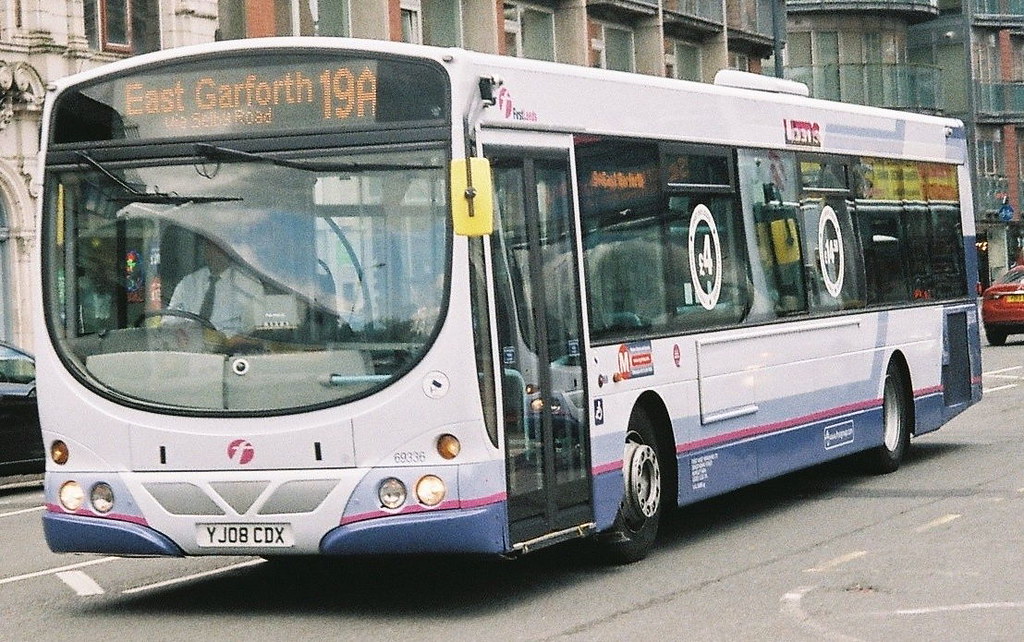The image depicts a large public bus in a closeup shot, primarily showcasing its front and left side profile. The bus is predominantly white with a dark blue edge border along the bottom and a small pink line. Displayed above the windshield in yellow digital text, the sign reads "East Garforth 19A via Selby Road." The bus driver, partially visible through the large front window, is dressed in a white dress shirt and a blue necktie, although his face is obscured by reflections. The bus has multiple windows and a large glass door for passengers. The scene includes a gray street backdrop, with apartment buildings visible on the left side. Positioned behind the bus on the right side is a red car driving in the opposite direction. The license plate YJ08 CDX is visible at the front of the bus.